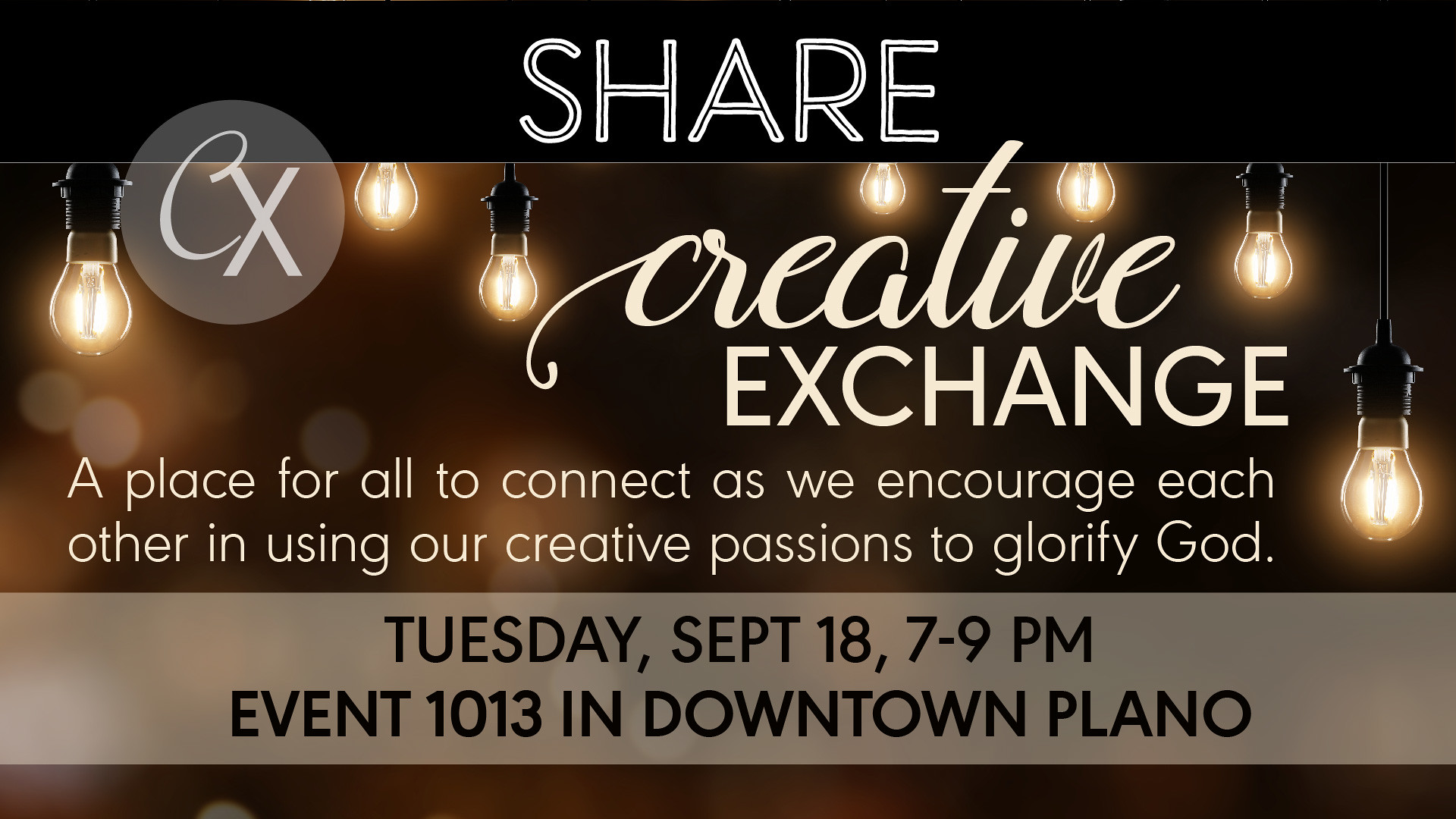The image is a wide rectangular advertisement with a prominent black header spanning the top fourth of the picture. Centered in white print on this banner is the word "SHARE," each letter defined by black highlights. Just beneath the header, an array of hanging light bulbs creates a striking visual, with some bulbs partially obscured by the header and others hanging down fully, revealing the cords they're suspended from. To the left, overlapping the header and extending downward, is a faded white circle containing the letters "CX." To the right, in a stylish lowercase cursive, the word "creative" is written, with "exchange" printed below it. Further down, about a third of the way from the left side, a message is presented in a light brownish-gray banner with black print, reading: "A place for all to connect as we encourage each other in using our creative passions to glorify God." Near the bottom of the image, another light-colored banner displays in black text: "Tuesday, September 18th, 7-9 PM, Event 1013 in Downtown Plano."